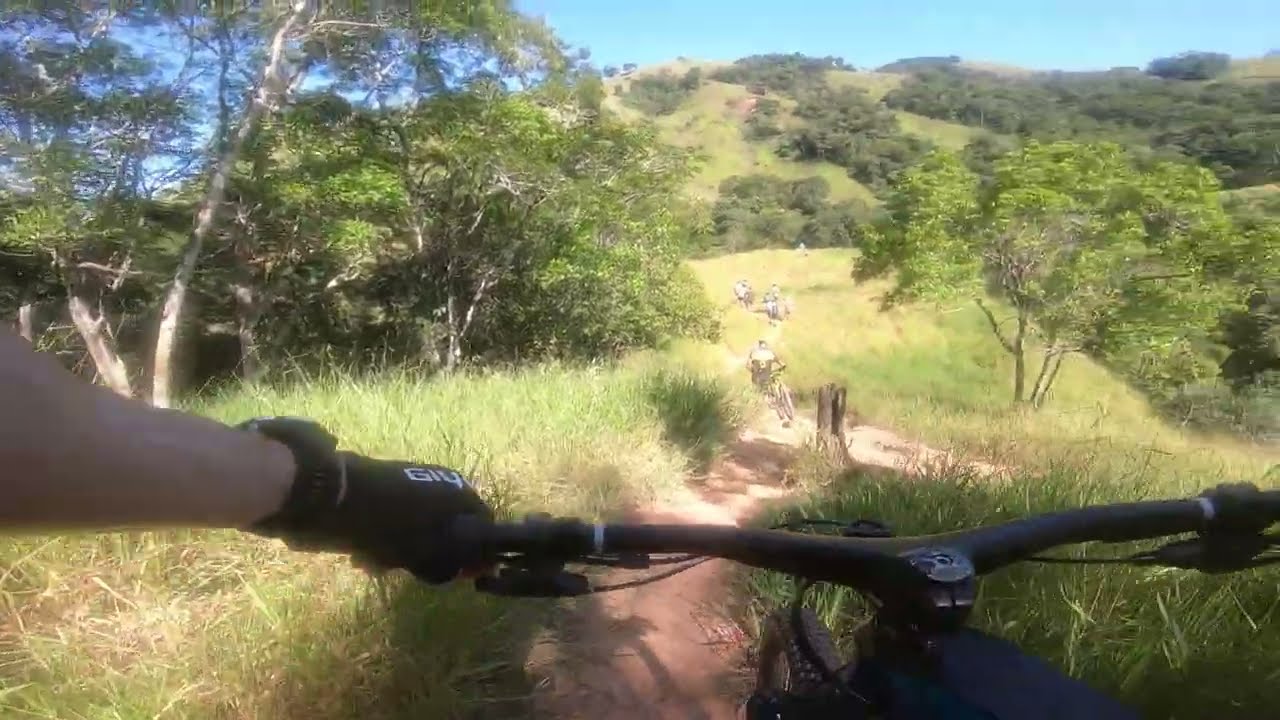The image captures a thrilling outdoor scene from the perspective of a mountain biker, likely using a helmet cam given the blurred motion, suggesting they are in action. The trail, a reddish-brown dirt path, descends steeply, indicating significant elevation loss. Tall grass, approximately two to three feet high, flanks the sides of this narrow trail. The path is bustling with activity, featuring several other mountain bikers, possibly partaking in a race. The biker’s left arm, clad in a black glove and possibly a wristwatch, grips the handlebar, with the bare forearm suggesting a Caucasian individual. In the distance, the landscape reveals undulating hills and patches of trees, painting a vibrant, wild terrain. The blue sky peeks from behind the hills, hinting at a clear daytime setting, enhancing the sense of adventure and the natural beauty of the scene.